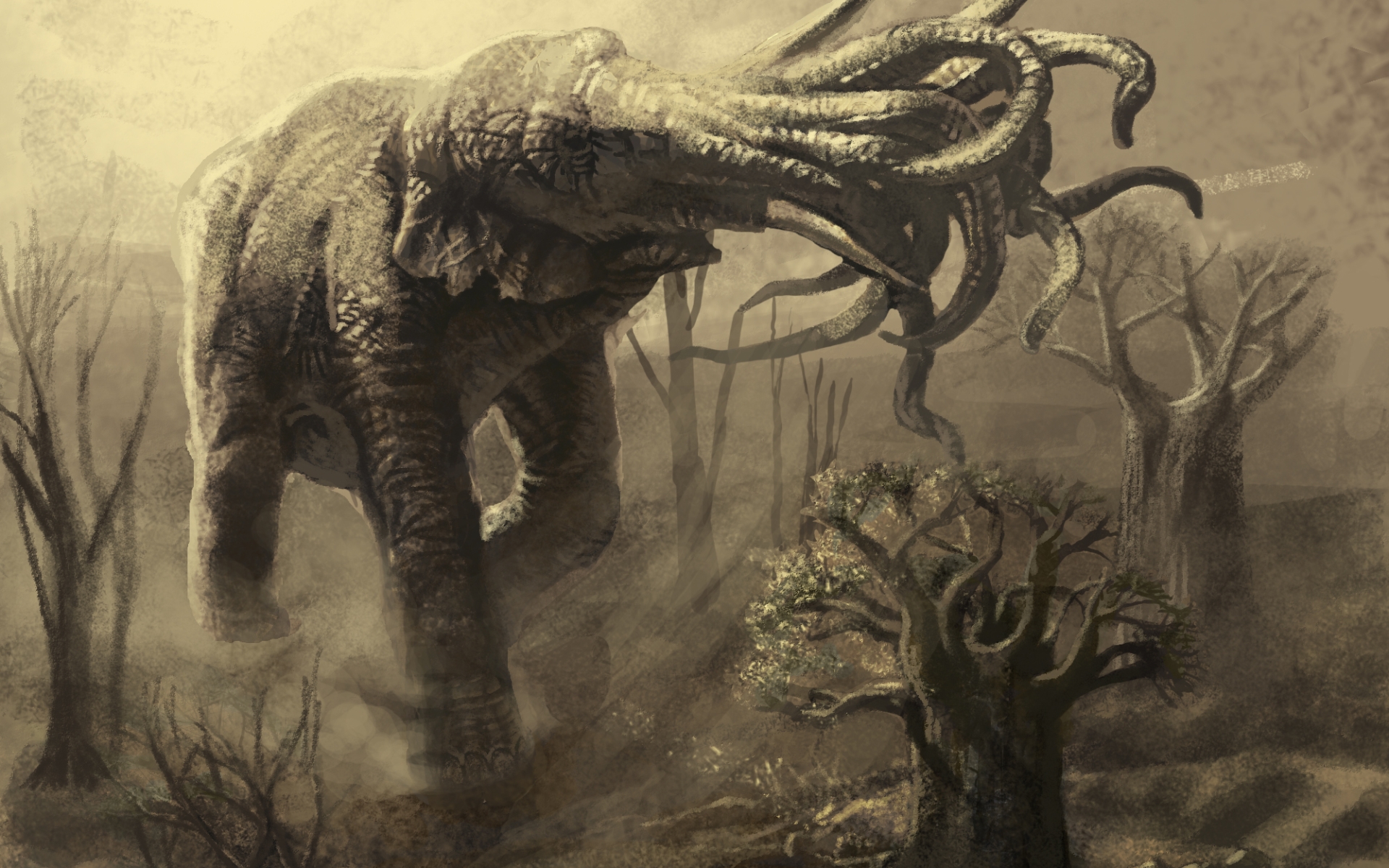This black-and-white illustration features a fantastical creature resembling an elephant with some sci-fi elements. The main subject is an enormous woolly mammoth-like figure, distinct for having numerous tentacle-like trunks, reminiscent of an octopus, sprouting from its forehead. It also has prominent tusks. The creature dominates a hazy, foggy forest landscape with small trees and short stumps scattered around. The background is rendered in various shades of gray, enhancing the eerie and otherworldly atmosphere of the horizontal composition.